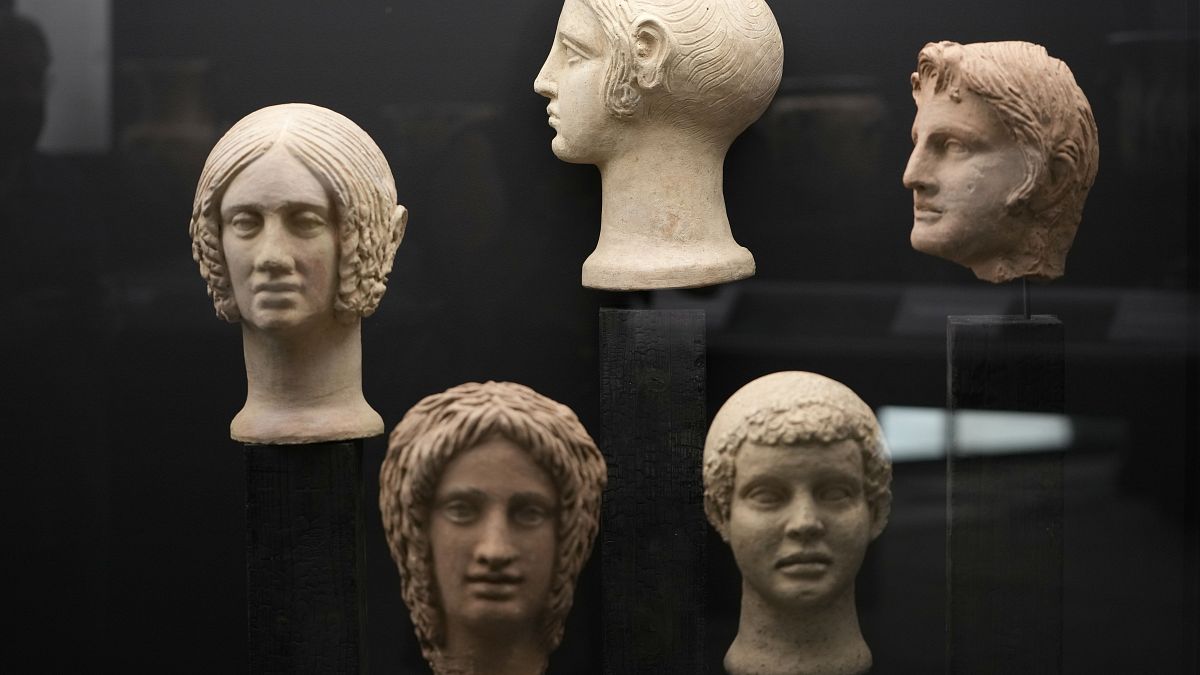The image is a color photograph in landscape orientation, depicting five sculpted head figures against a dark, almost shadowed, black background. The heads are arranged at varying heights, possibly mounted on clear plastic frames or shelves, and supported by black rectangular stands with slender poles.

In the center top of the image, there is a Grecian-style profile facing left. This figure has a distinctive curl of hair around the side of its head and an unusual back of the head formation resembling sideburns. To its left, in the middle row, there is another head with braided hair on both sides of its face, pointing upwards.

Directly below are two heads on the bottom row. The one on the left depicts a woman with long, flowing hair that hangs down the sides of her face. The head next to it on the right portrays a young boy with a modern, choppy hairstyle, sculpted in a light-colored stone that appears almost white.

Finally, on the top right, there's another profile of a Grecian-style face. This older man has defined features and is looking left, contrasting with the other heads’ varying styles and ages. Together, these sculptures form a circular, staggered formation, creating a visually striking representation of different historical and stylistic elements in sculptural art.